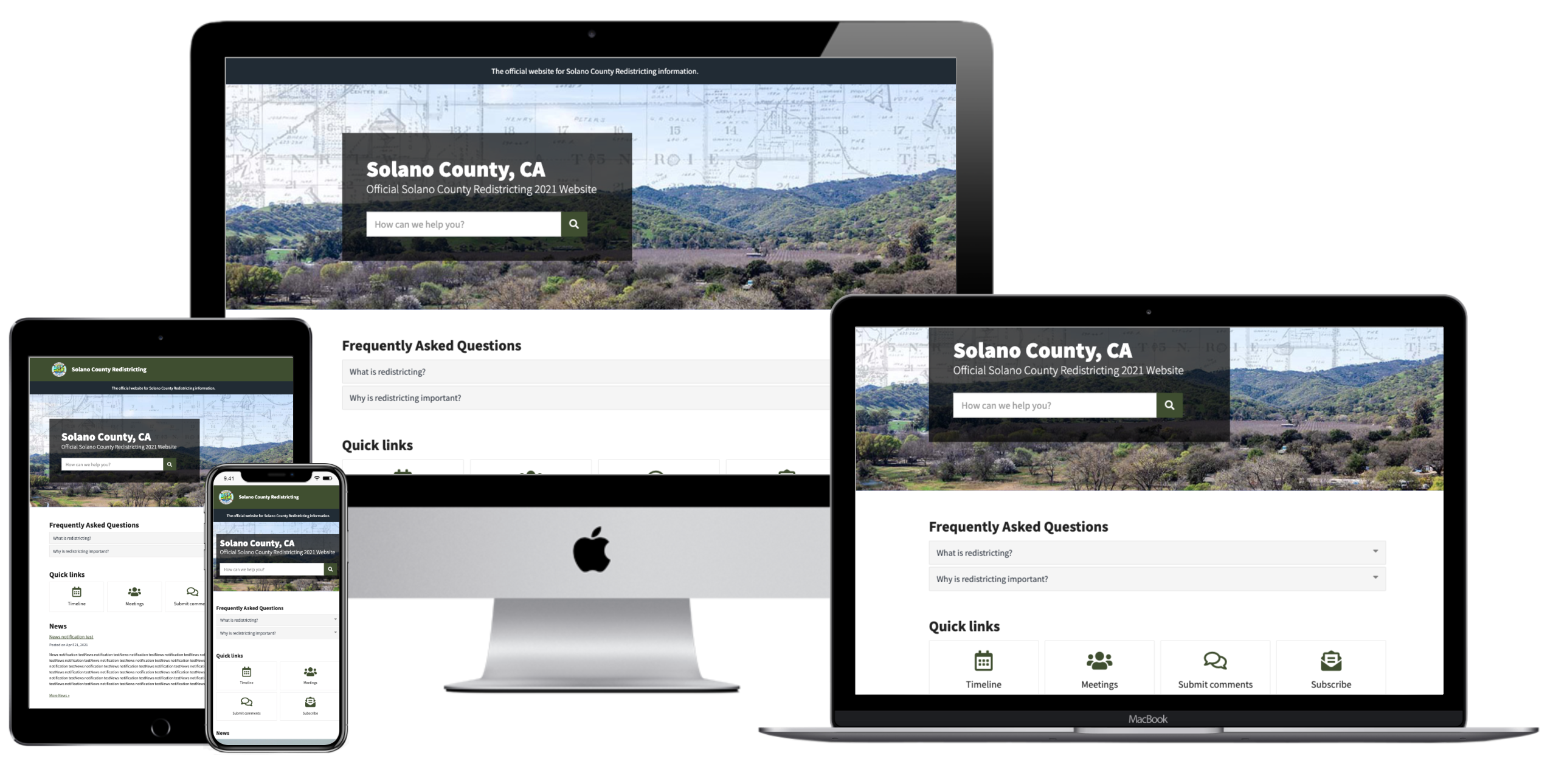In the image, there is a collection of Apple devices displaying the Salino County, California website. At the back, prominently featured, is an Apple monitor, showcasing the website with components such as a search bar, frequently asked questions, and a gray section labeled "Quick Links." 

In front of the monitor, a laptop presents the same website, maintaining all the details and features visible on the larger screen. 

To the right of the laptop, an iPad displays the website in a more vertical and condensed format, showing fewer elements of the page and consolidating the content. 

Lastly, an iPhone at the forefront shows a significantly minimized and cropped version of the website, displaying only a small portion of the content visible on the larger devices.

The Apple logo is distinctly visible on the base of the silver monitor, while the other devices, although not explicitly marked, are presumed to be Apple products due to their similarity in design and the cohesive grouping.